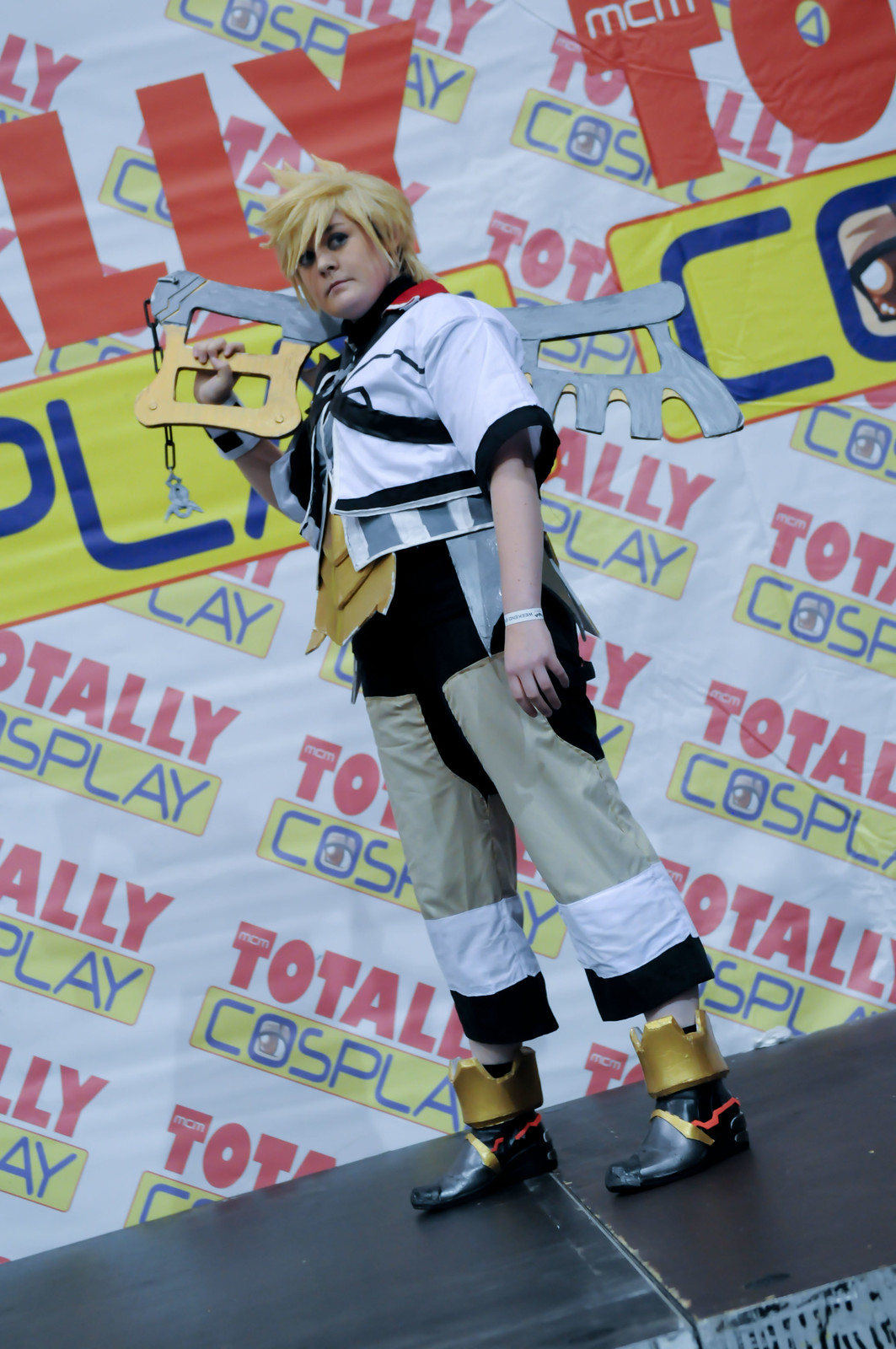The image depicts a cosplayer, possibly a woman, standing confidently on a black platform in front of a large, brightly lit backboard that reads "Totally Cosplay." The person is dressed in a detailed cosplay outfit featuring a distinctive blonde wig and an intricately designed ensemble of white, black, gray, and beige, complemented by black and gold boots. The outfit draws elements from various sources, including a karate-style suit with black and white trim and a faux metal belt. Over their right shoulder, they are holding a large, intricate weapon or key, adding to the dramatic and elaborate nature of the costume. The scene is bathed in natural light, enhancing the clarity and vivacity of the colors, and the person strikes a pose that suggests they are deeply immersed in their character. There are no other individuals in the photo, which focuses solely on the cosplayer and their detailed, eye-catching attire.